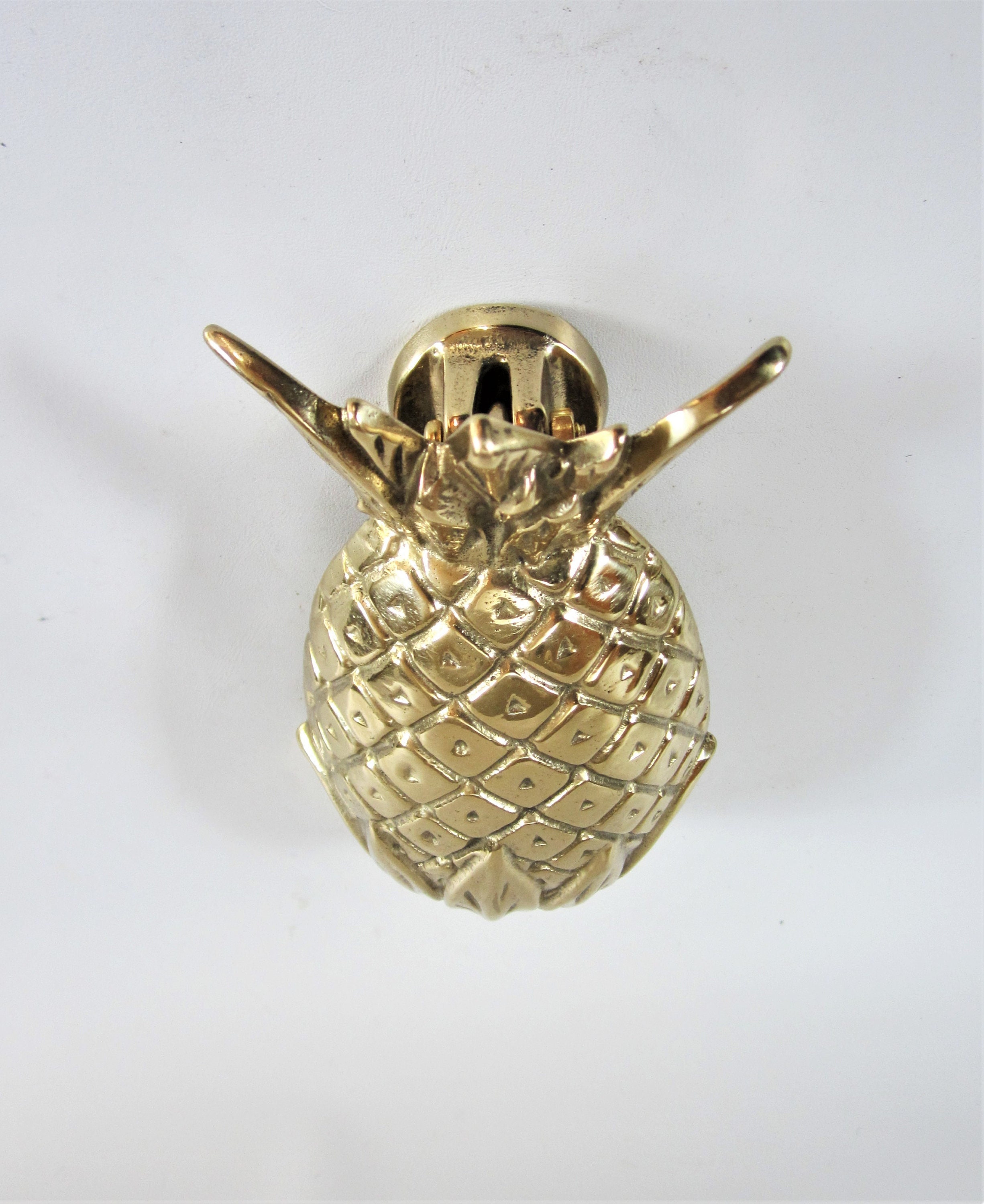The image captures a detailed photograph of a golden pineapple pin or brooch, sharply set against a stark white background. The pineapple, exquisitely crafted to near perfection, boasts intricate, engraved diamond patterns with small indentations in the center of each diamond, enhancing its lifelike appearance. The solid gold leaves of the pineapple, engraved at both the top and bottom, extend outward and shimmer with a mirror-like finish, despite bearing slight imperfections like metal smudges and scratches toward the upper section below the leaves. Although primarily intended to showcase the front of the pineapple, the photo angle downwards reveals the fastening mechanism on the back, drawing attention to the clasp and somewhat diverting focus from the head-on view of the pristine golden surface.